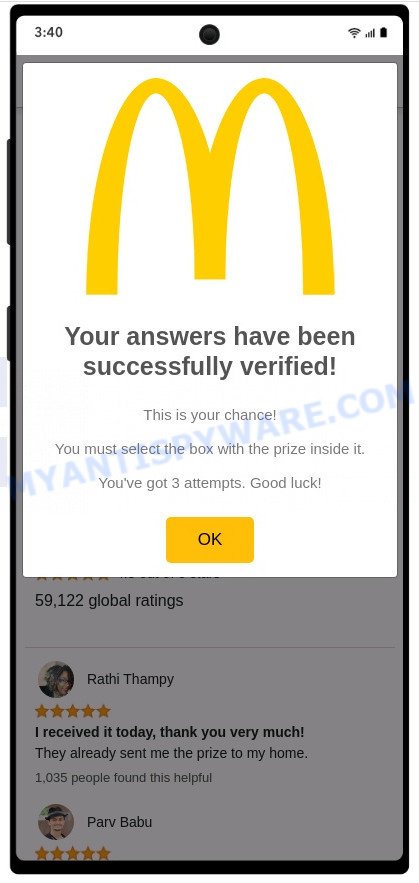Screenshot from an Android Phone Displaying a McDonald's Promotional Message

The image is a screenshot taken on an Android smartphone, evidenced by the distinctive circle in the middle of the top bar housing the front camera. The status bar at the top displays the time, Wi-Fi signal strength, network signal, and battery percentage, reflecting typical Android features.

Beneath the status bar, a large yellow "M" logo, representing McDonald's, is prominently displayed. Below the logo in bold black letters, the text reads: "Your answers have been successfully verified." Further down in smaller black letters, the message continues: "This is your chance. You must select the box with the prize inside it. You've got three attempts. Good luck."

A yellow button with the word "OK" in black letters is positioned below the text, prompting user interaction. This entire message is overlaid on another page.

The underlying page features user reviews. One review, by a user named Rathi Tharnpe, includes an avatar of a black woman with dark black hair. Rathi gives a five-star rating and states in bold letters, "I received it today. Thank you very much." Below, she further comments, "They already sent me the prize to my home," with 1,035 people finding her review helpful.

Another review shows the profile of a white man wearing a black hat, named Par Babu, who also gives a five-star rating. Between the two reviews, a metric indicates "59,122 global ratings."

This image captures a promotional message from McDonald's, encouraging user participation, with a backdrop of user reviews attesting to successful prize reception.